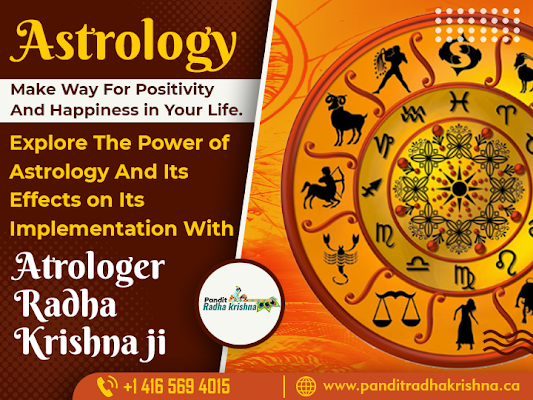The image is an advertisement for an astrology business featuring a split background with a gradient of dark to light orange diagonally divided. On the right side, there's a prominent circular wheel displaying various zodiac signs, each illustrated with their respective animal symbols—like fish for Pisces, ram for Aries, and scorpion for Scorpio—encircling a central sun icon, forming an astrology chart. On the left side of the image, the text "Astrology" is written in yellow font, accompanied by a motivational phrase in brown font on a white background: "Make way for positivity and happiness in your life." Below that, on a brown background with yellow font, it states: "Explore the power of astrology and its effects on implementation with," followed by "Astrologer Radhakrishnaji" in white font. At the bottom of the image, additional contact information is provided, including a phone number, "+1-416-569-4015," and a website, "www.panditradhakrishna.ca." A white circle on the right side also mentions "Pandit Radhakrishna."